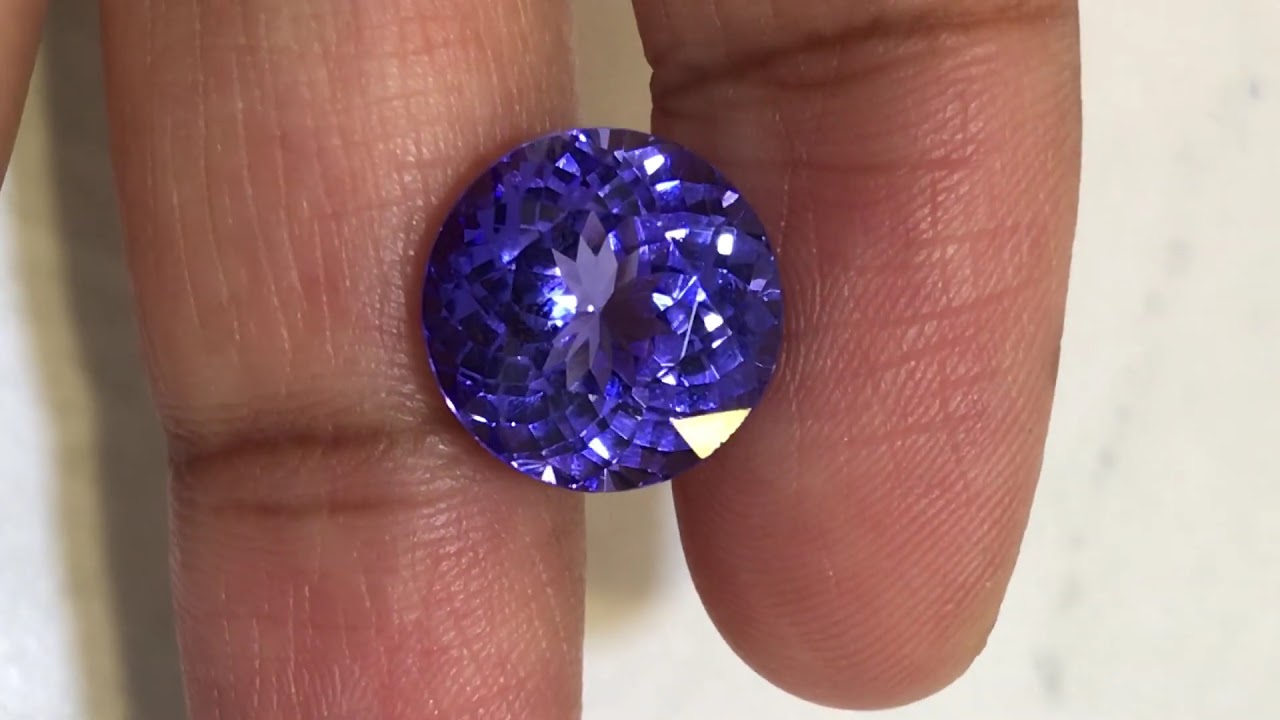This close-up image showcases the tips of two fingers delicately holding a vibrant, circular blue gemstone. The gem, approximately the size of a dime, exhibits a mesmerizing bluish-purple hue with facets that reflect light, giving it a glowing appearance. The intricate cuts on the gemstone create numerous small squares and triangles, contributing to its radiant sparkle. In the center of the gemstone, a pattern resembling a white, leaf-like figure emerges, reminiscent of a flower, although this design is not explicitly carved or printed. The skin on the fingers reveals horizontal lines and finer vertical indents, indicating the natural texture of human hands. The background is a plain white, ensuring full attention is directed towards the captivating blue gemstone and the carefully holding fingers.